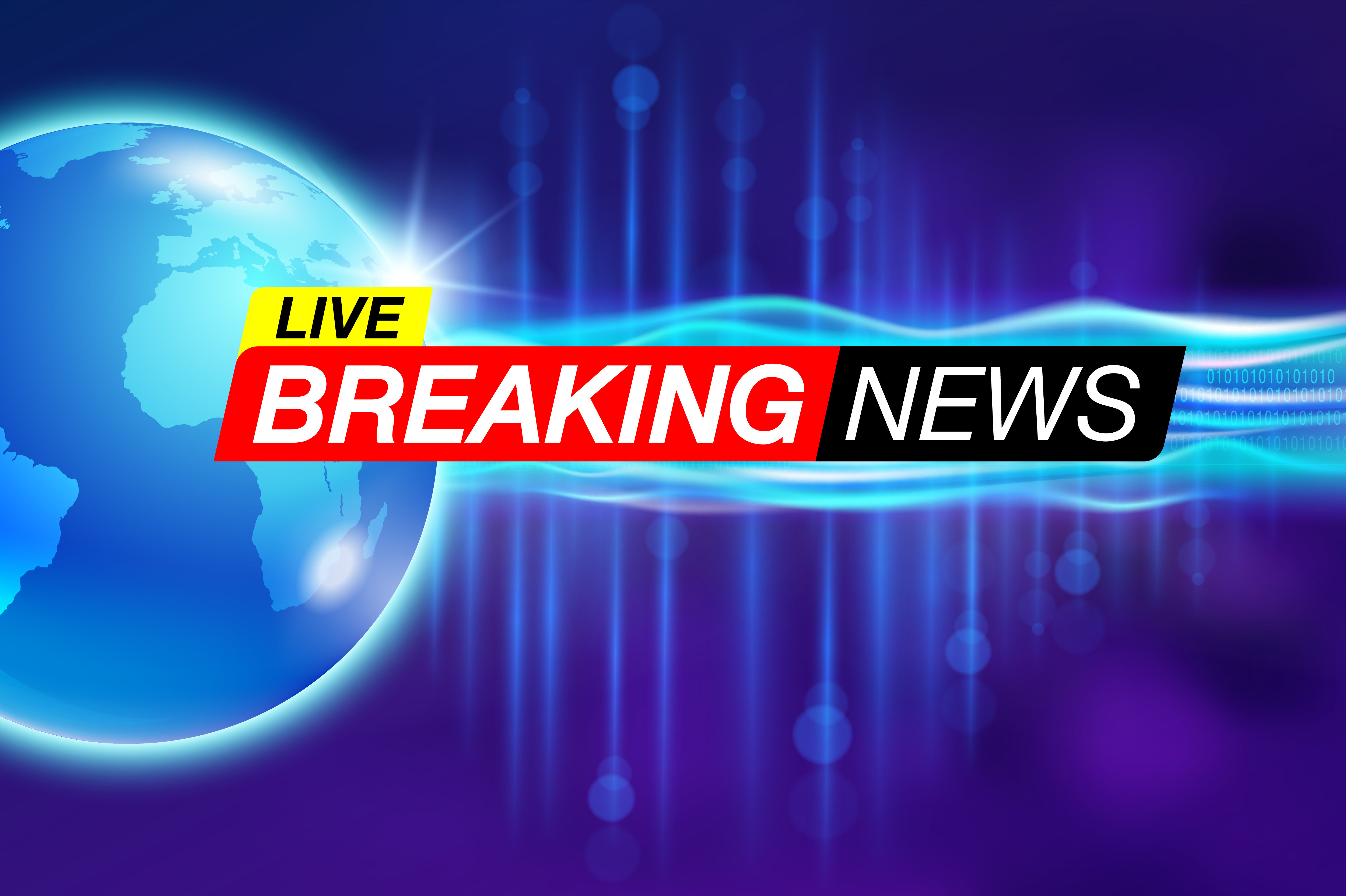The digital illustration features a dark blue and dark purple background that seamlessly blends into a deep, atmospheric backdrop. On the left side is a glowing, turquoise-blue globe emitting bright, wavy lines that extend to the right. Central to the image is a yellow parallelogram with the word "LIVE" in bold text, flanked below by a red rectangle with "BREAKING" in white, large-font lettering. To the right of this red rectangle, a black parallelogram contains the word "NEWS" in a similarly large font. The composition is accentuated by blue, sound-wave-like lines cutting horizontally across the scene, along with repeating digits "100100," adding a cryptic digital element.